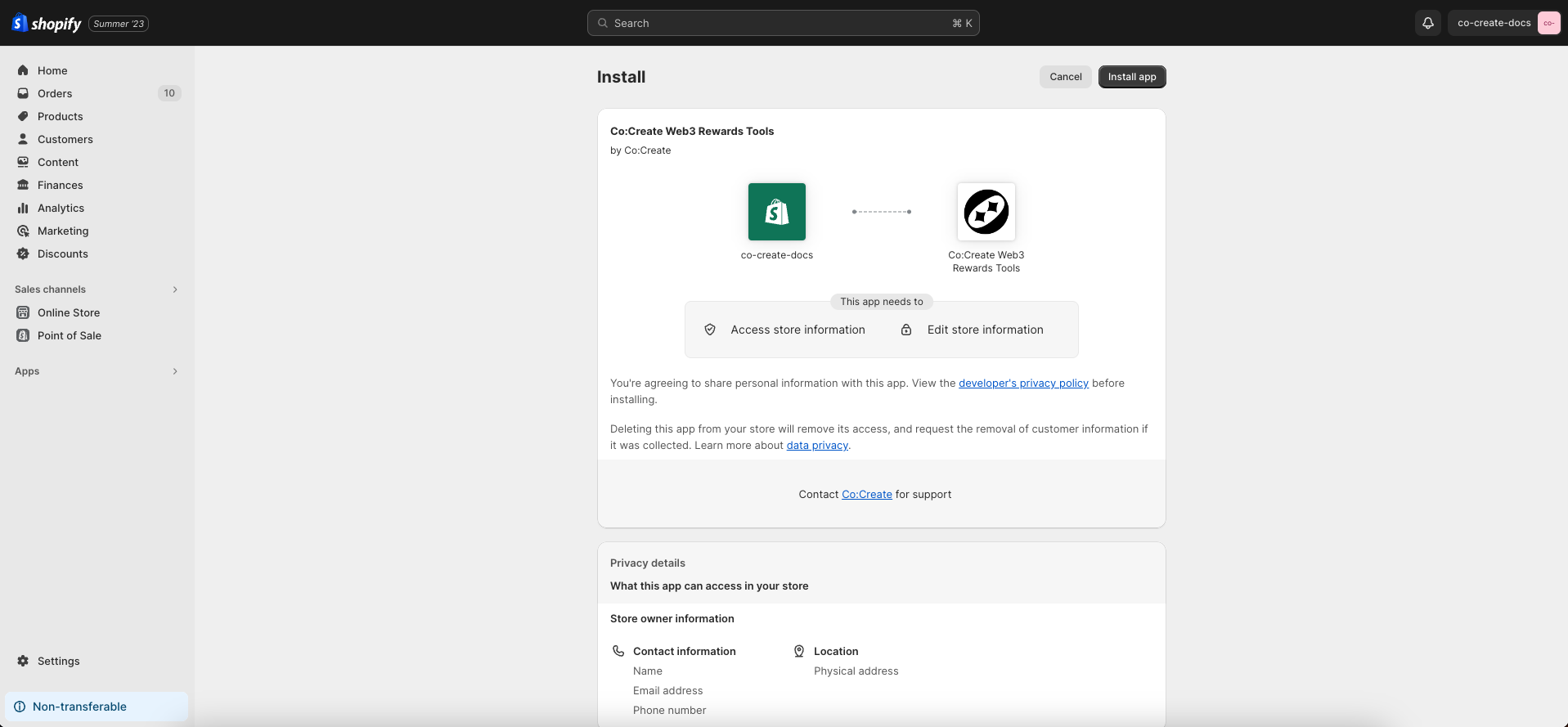This landscape screenshot, likely taken from a laptop, features the Shopify dashboard. A prominent black stripe spans the upper left to upper right sections, with the Shopify logo and name on the upper left. Adjacent to this, within a circle, is the text "Summer '23." Centrally located in the top section is a search bar, while the upper right corner contains a notification icon followed by the text "co-create-docs."

The main section beneath the header is split into two distinct columns. The left sidebar, which acts as a navigation menu, lists options as follows: Home, Orders (with a notification indicating 10 new orders), Products, Customers, Content, Finances, Analytics, Marketing, Discounts, and Sales Channels. The Sales Channels submenu includes Online Store, Point-of-Sale, and Apps. At the sidebar's bottom, there is a 'Settings' option and a blue button labeled 'Non-transferable.'

The right-side column of this section, which has a slightly lighter gray background, includes a header that says "Install" and a top-right 'Cancel' button. Below, a black 'Install App' button is prominently displayed. The body of this column features a large white area with the text "Co-create Web 3 Rewards Tool by Co-create." This section explains that the app, co-create-docs, will interact with "Co-create Web 3 Rewards Tool" and needs access to store information for editing purposes.

Further down, there are hyperlinks included for user awareness and consent. These include agreeing to share personal information with the app, (viewable via a link to the developer's privacy policy) and a 'Data Privacy' policy link. Lastly, there is another blue hyperlink related to Co-create at the very bottom of this column.

Overall, this detailed screenshot provides comprehensive navigation and app installation instructions within the Shopify platform.